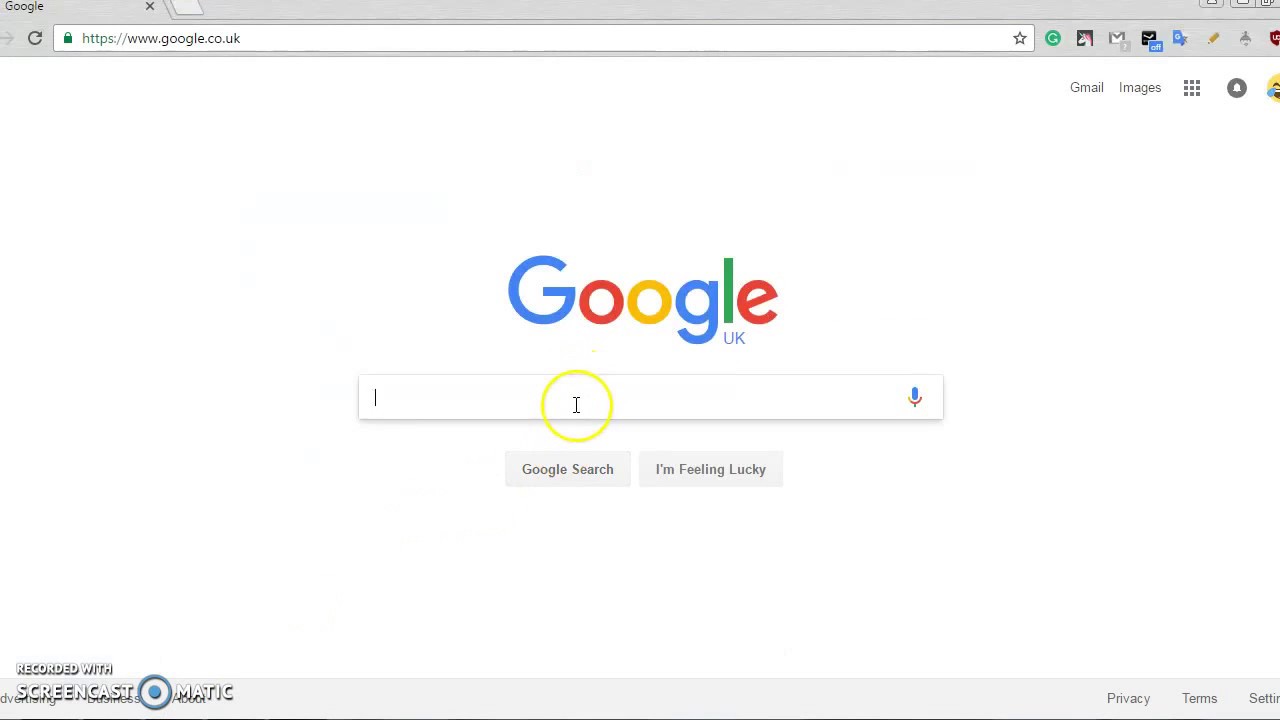The image showcases the Google homepage with the URL www.google.co.uk. The entire background is white, creating a clean and simple interface. 

At the top-right corner, options such as Gmail, Images, an App icon, and a Notification icon are listed in grey text, providing easy access to various Google services.

Centrally positioned is the iconic "Google UK" logo. The "G" is blue, the first "o" is red, the second "o" is yellow, the "g" is blue, the "l" is green, and the "e" is red. Below the "L," there is a small, purple "UK" signifying the localized version of the site.

Beneath the logo is the search box, also white. To its right, there is a microphone icon adorned with Google’s signature colors. Inside the search box, there is a yellow cursor indicating the user is engaged in typing.

Below the search bar are two grey buttons for search functions: "Google Search" on the left and "I'm Feeling Lucky" on the right.

At the bottom-right of the page are footer tabs labeled Privacy, Terms, and Settings, while the bottom-left contains links for Advertising, Business, and About. 

Above these left-side tabs, there's a watermark reading "Recorded with Screencast-O-Matic." The text is vertically aligned, with "Screencast" at the top and "Matic" at the bottom, separated by a blue circle with a darker blue inner circle.

This detailed description captures all visual elements and their placements on the Google UK homepage depicted in the image.